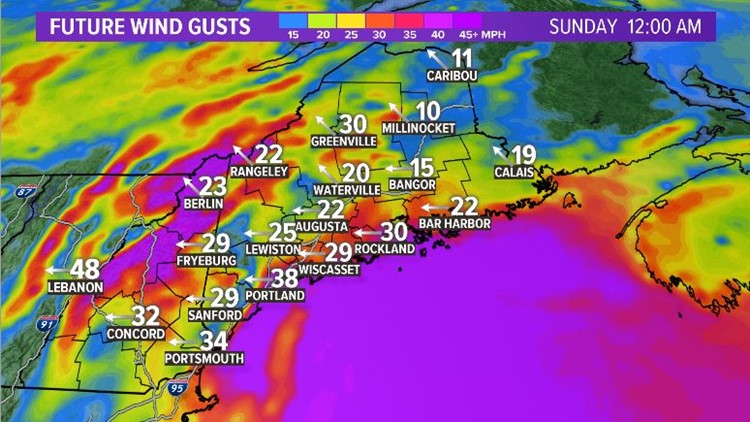This detailed weather map focuses on the anticipated wind gusts for the New England area of the United States, specifically around the state of Maine. At the top of the map, a thin purple-indigo bar labeled "Future Wind Gusts" serves as a color key, translating colors to wind speeds ranging from 15 to 45+ miles per hour. The map is timestamped for Sunday at 12 a.m., and it is marked with various colors representing different wind speeds: blues and greens for lower speeds, yellows and oranges for moderate speeds, and pinks and purples for the highest speeds. On the map, notable cities such as Portland with 38 mph winds and Bar Harbor with 22 mph winds are highlighted. Each city also features a directional arrow indicating the expected wind direction. The highest speed recorded is 48 mph. This vibrant and detailed map allows for a clear understanding of the wind gust predictions, essential for making informed decisions about the upcoming weather conditions.